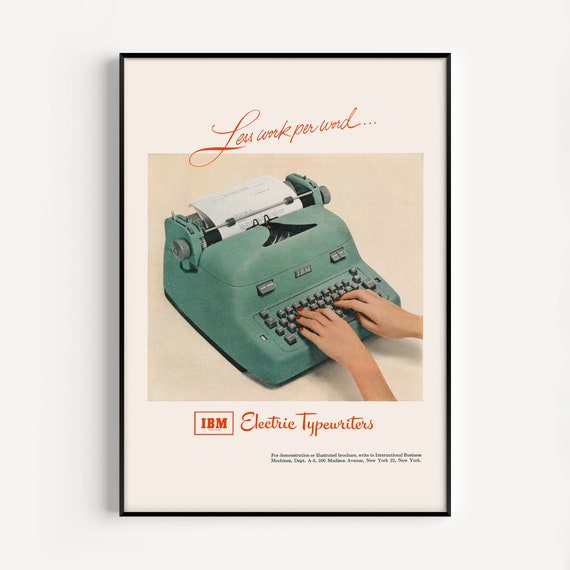The image depicts a framed poster from the 1950s featuring an IBM electric typewriter. The poster is predominantly white with red text and a black frame. Central to the poster is a photograph of a woman typing on a light green, or aqua-colored, IBM typewriter. The text above the photograph reads "Less Work Per Word..." and below it, alongside the IBM logo, are the words "electric typewriters." The setting suggests a mid-20th century advertisement with a nostalgic, vintage aesthetic. The background outside the poster is a muted grayish whiteness, giving a stark contrast to the lively colors within the frame.